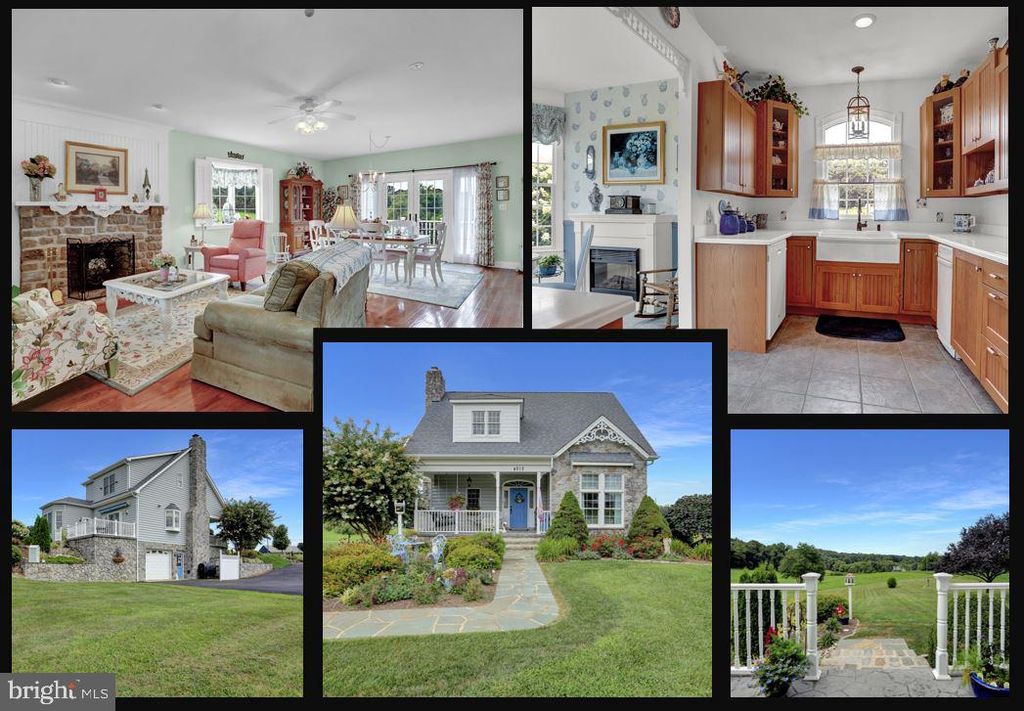This landscape-mode, color photograph is a composite image featuring five different images of the same property, styled like a real estate advertisement. Dominating the bottom center is the main photo of a charming two-story house with a mixed stone and wood exterior. The home is set on a beautifully manicured lawn that wraps around the property, which spans over an acre. The exterior features a clean, 90-degree stone pathway lined with medium-sized shrubs and flower gardens, leading up to the front entrance.

The house is a quaint farm-style home with a gray exterior, attached garage, and approximately eight front windows, including a chimney made of gray rock. Inside, the house reveals a blend of vintage and modern decor. The living room, featured at the top left of the composite image, has country-style white and beige tones, a fireplace, a mantel adorned with lace and tchotchkes, and a beige couch covered in white fabric.

The kitchen is equipped with brown wooden cabinets, white countertops, and a white tile floor, with additional details like white walls and white wallpaper. Despite its modern furnishings, including a dining room table and colorful decor with bright whites, greens, and blues, elements like the lace on the mantel suggest an older resident's touch. Flower gardens and a spacious, verdant yard add to the overall idyllic and inviting ambiance of this picturesque property.